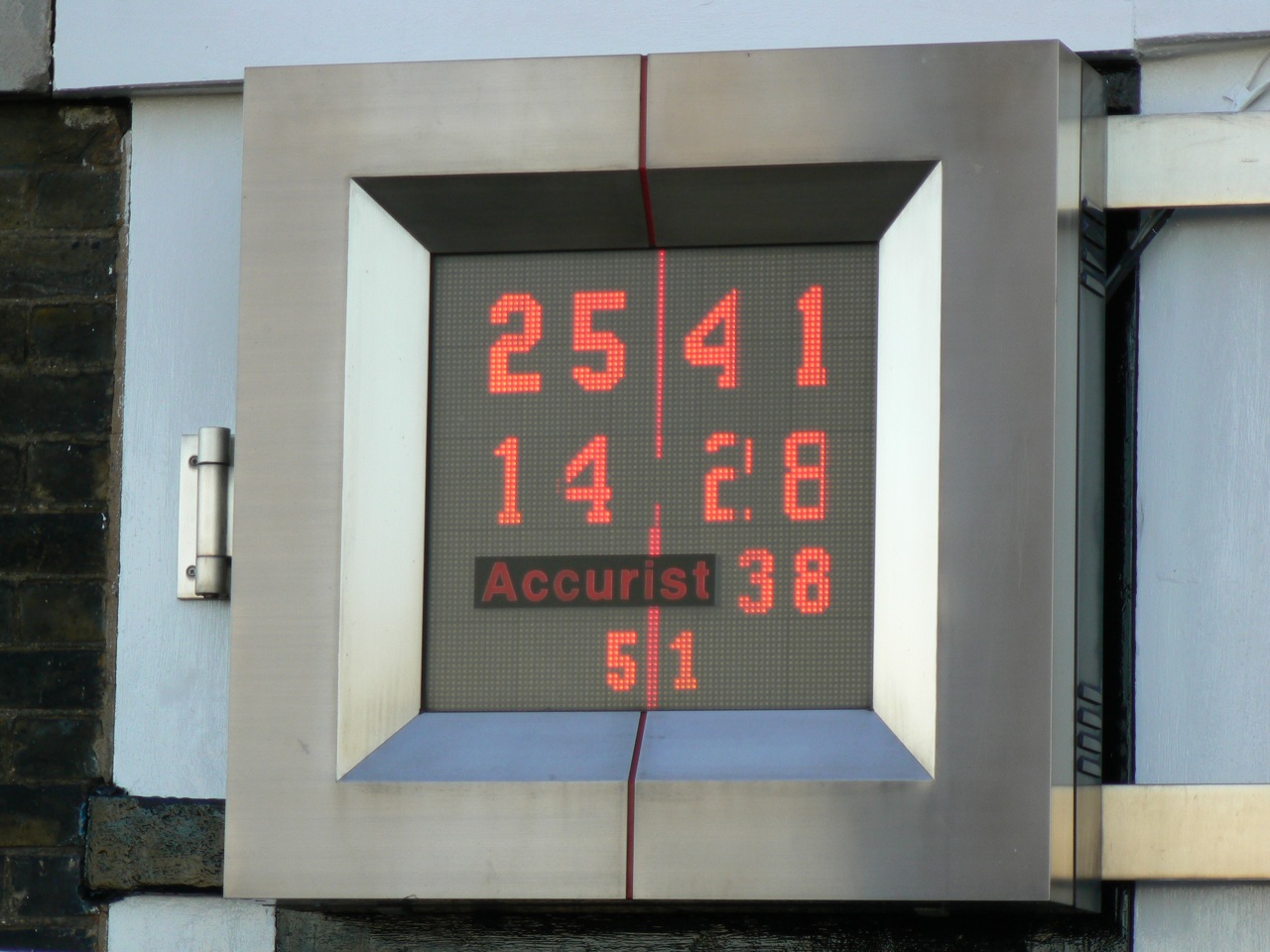The image depicts a brick building featuring an architectural element that might either be a window or an inset panel. Prominently built into the structure is a digital sign, framed by a substantial stainless steel border that creates a C-shape on the left and a mirrored, backward C-shape on the right. The metallic borders extend around the sign but do not complete a full enclosure, leaving a distinct gap in the middle.

The sign's border is hinged on the left-hand side, suggesting possible functionality for maintenance or access. The digital display exhibits the name "Acurist," likely indicating the manufacturer or sponsor of the sign. The sign itself is divided into sections with various numbers displayed. On the left side, the numbers "2-5" and "14" are illuminated. On the right side, from top to bottom, the numbers "4-1," "2-8," and "38" are shown, with the latter being in smaller digits. Additionally, there is a "5" and a "1" displayed at the very bottom on each side. The purpose of these numbers is unclear, leaving their significance open to interpretation.